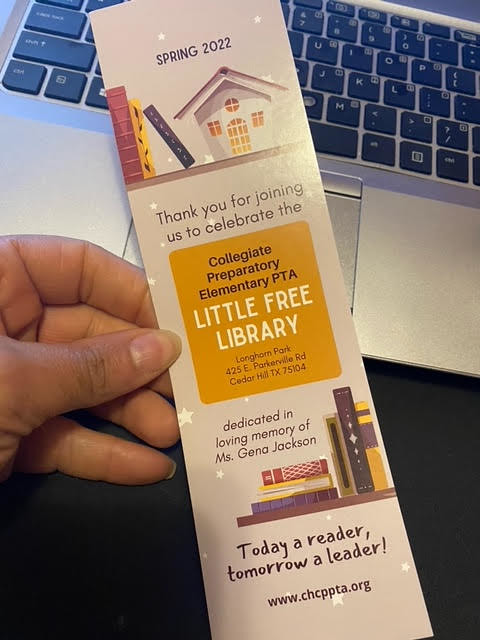The image is a vertically aligned, color photograph taken in portrait orientation, featuring a person's hand holding a printed bookmark over a silver MacBook keyboard. The background shows the keyboard with black keys and white letters, and a black desk beneath the laptop. The hand, positioned on the left side of the image, appears to be a female's left hand with a long, curved thumbnail and light brown skin.

The white bookmark, held centrally in the image, is topped with the text "Spring 2022" in blue letters. Below this, there is an illustration of a white cottage beside a stack of colorful books. The text under the illustration reads: "Thank you for joining us to celebrate the," followed by a prominent yellow square containing the words "Collegiate Preparatory Elementary PTA, Little Free Library," and the address: "Lone Hand Park, 425 E Plainwelled Road, Cedar Hill, Texas 75104." Further down, the text "Dedicated in loving memory of Ms. Gina Jackson" is inscribed, accompanied by another image of books. At the very bottom, the slogan "Today a reader, tomorrow a leader!" and the URL "www.chppta.org" are displayed.